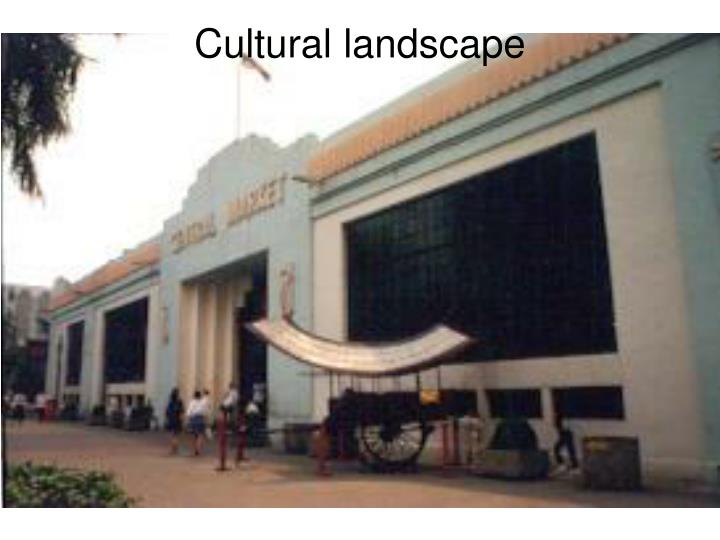This color photograph, although quite out of focus, captures the front of a very large, tall building with the word "market" prominently displayed across its top. The edifice appears to be made of stone with a white facade, accented with a terracotta and green border along the top, and features a tall flagpole. The scene suggests it may be located in a cultural landscape, possibly in Mexico, based on its architectural style and the "cultural landscape" text overlaid in black at the top of the image. In front of the building stands an old-fashioned wooden cart with large wooden spoked wheels and a metal, canopy-like roof. The cart is cordoned off with ropes and poles, indicating that it is not accessible. The area appears to have cobblestone streets, and several people dressed in white shirts are seen walking towards the building, adding a sense of activity to the blurred historical ambiance of the photograph.